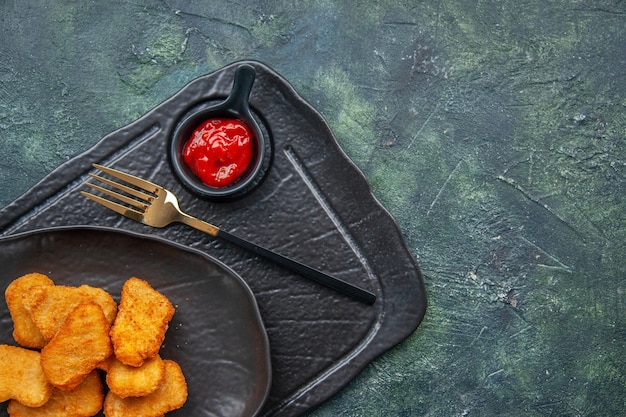This is a detailed close-up food photograph featuring a sophisticated layout. The focal point is a black plate, centered on an elegant black Art Deco tray. On the plate, we see golden brown chicken nuggets stacked appealingly. Adjacent to the nuggets, a silver fork with a black handle is strategically placed on the tray. The tray also includes a small serving dish with a handle, filled with bright red ketchup. The entire setting rests on a stylish grayish-blue stone table, showcasing a marbled effect with hints of dark gray and subtle light green tones. The stone surface appears slightly worn in a few places, adding character to the scene. The ketchup dish, nuggets, and fork are arranged artistically, creating a visually compelling and appetizing composition.